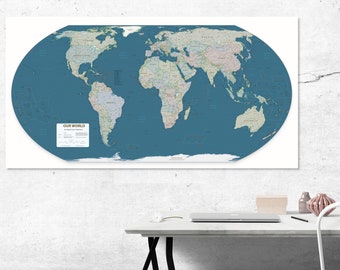The image features a large, prominently displayed map of the world, resembling a Mercator projection with straight lines at the top and bottom and curved edges. The map, predominantly in shades of blue and tan, is mounted on a white background, affixed to a primarily grayish-white wall. A noticeable crack runs down the right side of the wall. In the lower right-hand corner of the image, a desk with black legs supports a closed laptop, accompanied by a pen, two bottles in a gift box, and a couple of small knick-knacks, including what appears to be a white flower or earphones. A white chair is positioned in front of the desk, completing the scene.